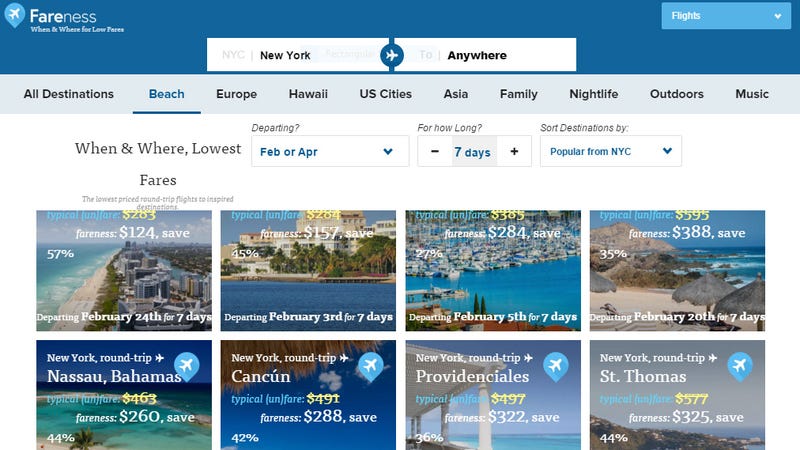This image captures a detailed web page interface designed for booking travel arrangements. In the top left corner, we see the interface for selecting "Fairness" and specifying the "When and Where" section for finding low fares. The destinations listed include options like New York, Seoul, and other locations across categories such as all destinations, beaches, Europe, Hawaii, US cities, Asia, family trips, nightlife, outdoor adventures, and music events. 

Users can specify their travel parameters, including "Lowest Fares" and departure timeframes like February through April, for trips lasting around 7 days. There is a highlighted deal indicating a popular destination from New York City, departing on February 24th for a 7-day trip, with a fare of $124, reflecting a 57% sale.

The webpage is visually appealing with colors like blue, white, and yellow, contributing to a pleasant user experience. The image also includes snapshots of various cities and scenic ocean views, perfect beaches, enhancing the sense of wanderlust and travel inspiration for potential bookers.